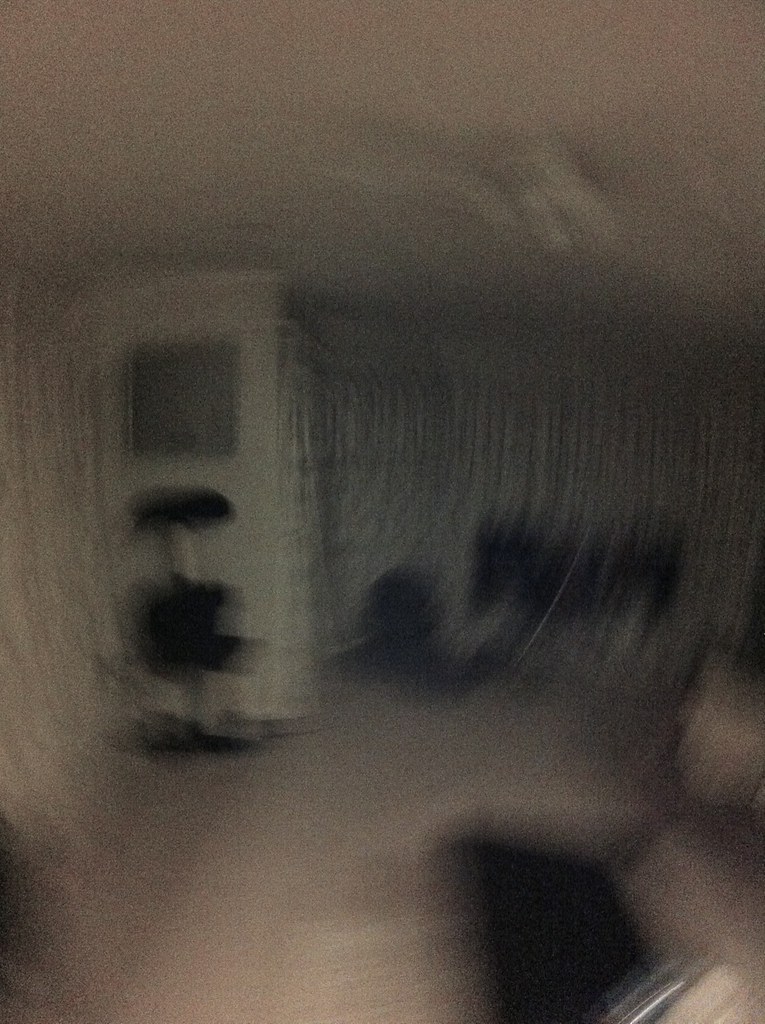This indoor color photograph is extremely blurry, grainy, and dimly lit, making it difficult to distinguish details. The scene appears to be a room with a light white ceiling and a light tan floor. Central to left of center, there is a large white wall or a door, possibly with a top window, and in front of it stands what might be a black chair or exercise equipment like a stationary bike with a black seat and console. On the right side of the image, in the background, there are vague black shapes that could be more exercise equipment or furniture. A black-gloved hand is vaguely visible at the bottom right, and the overall scene is enveloped in shades of gray and a dusty rose hue. The photograph’s blurred and grainy appearance, possibly due to being taken with an older camera that was jostled, provides an ambiguous atmosphere, leaving much to the imagination.